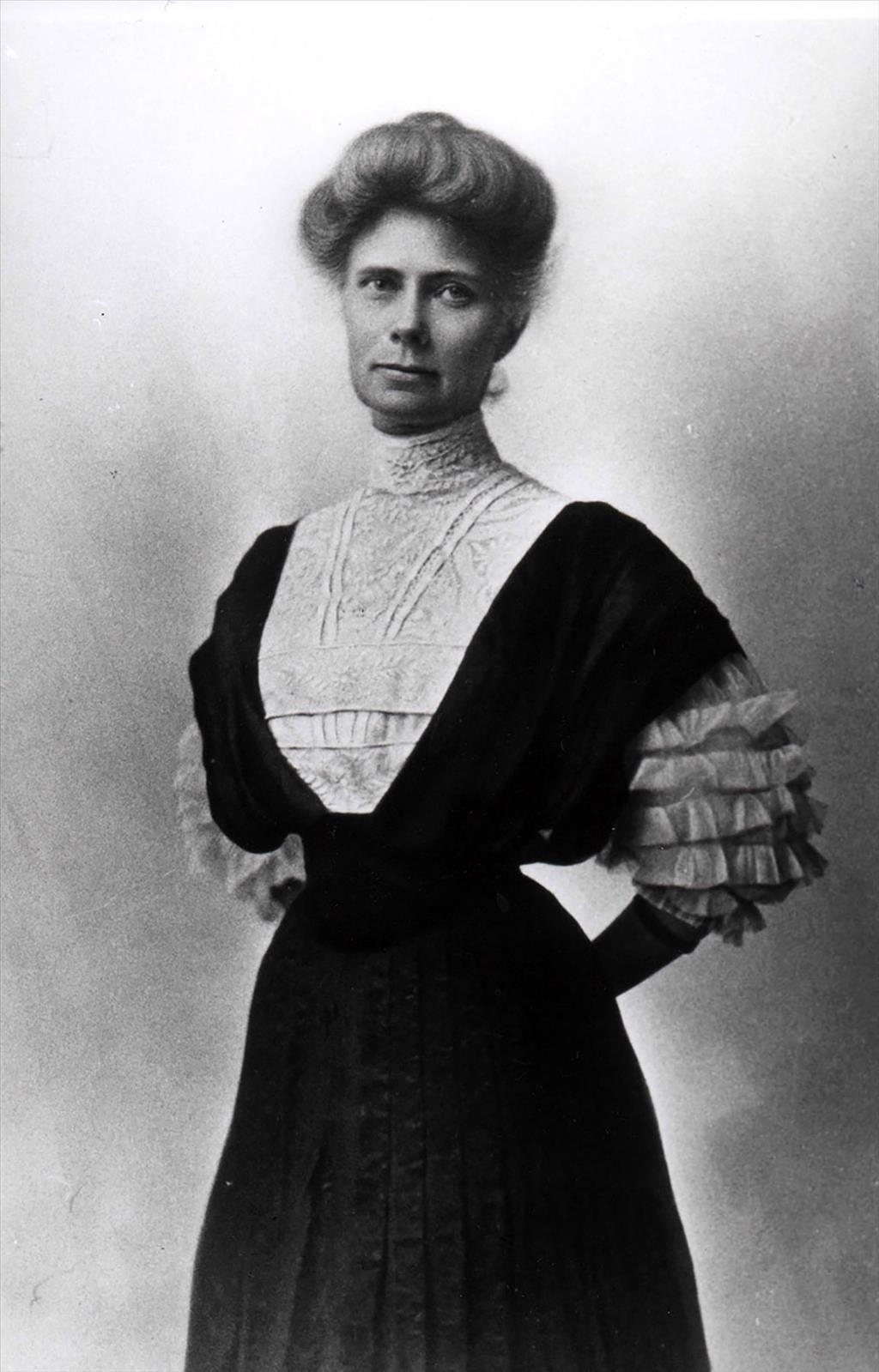This is an antique black and white photograph likely from the late 1800s or turn of the century. The image features a woman in her thirties positioned centrally. The background is a gradient of light to dark grays, and the photograph appears to have noise, dust, and scratches, suggesting it is either an original film negative or heavily processed. A notable white halo surrounds the woman, hinting at darkroom processing or AI enhancement. She is dressed in a long, black dress with white decorative fabrics in the center and fluffy, lighter colored short sleeves. Her hair is neatly styled in a bun. The woman's expression is subtle with a slight suggestion of a smile and well-trimmed hair. She gazes away from the camera, adding an air of mystery to the carefully staged studio portrait.